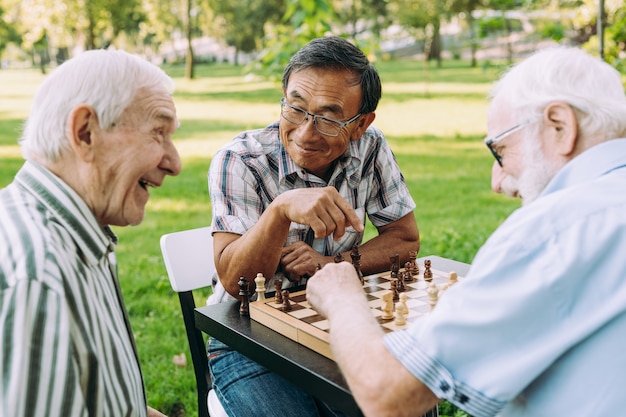The photo features three elderly men sitting outdoors around a small table, fully engaged in a game of chess. The scene is set in a park-like area with blurred green grass and trees in the background, dappled with sunlight and shadows. The man on the left, with strikingly white hair, is observing the game. He has a joyful expression, marked by his many wrinkles, and wears a green and white striped dress shirt. The man in the middle, who is darker-skinned and likely Asian, is actively participating in the game. He sports glasses and a gray striped shirt, holding a chess piece in his hand while glancing at the observer on his left. The man on the right, also playing chess, is focused on the board. He has white hair, glasses, and a light blue short-sleeved shirt. The wooden chessboard in front of them is a mix of teak color with black, brown, and white squares, supporting an array of corresponding chess pieces.